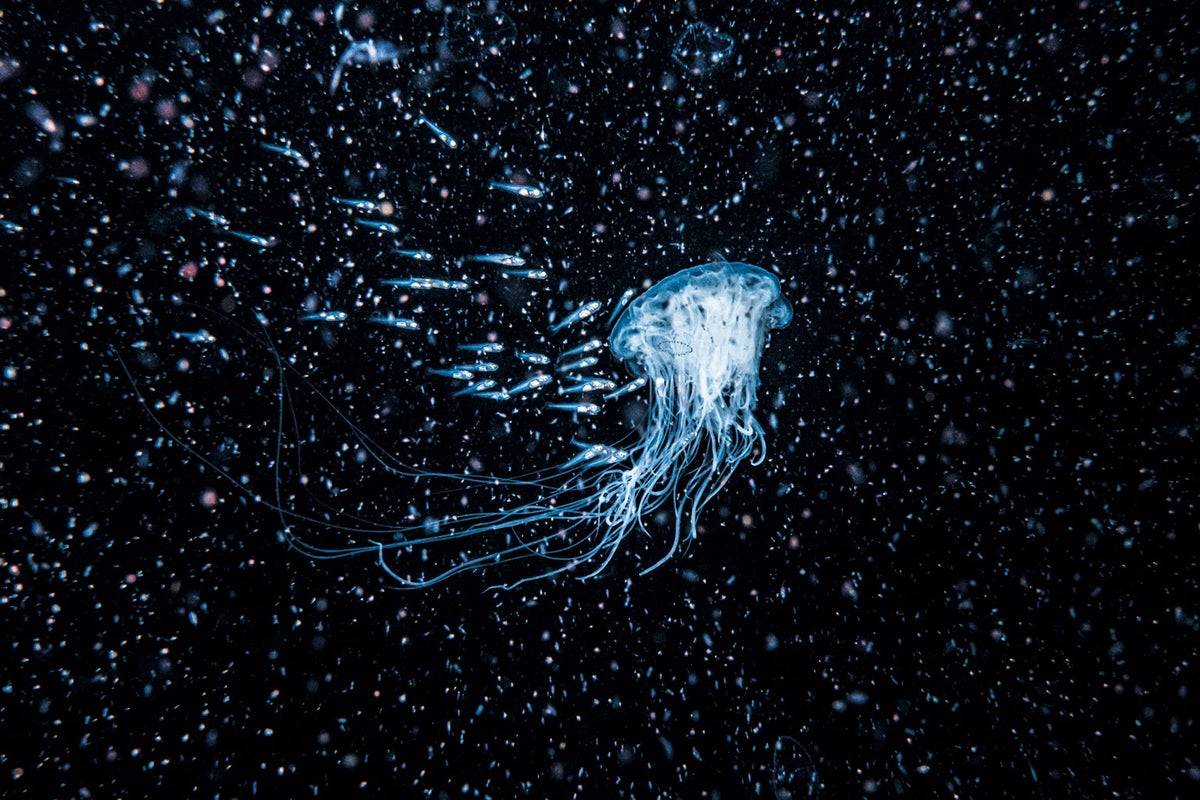This captivating horizontal rectangular image, initially reminiscent of a starry night sky, is actually an underwater photograph taken in deep, dark waters. At the center, a ghostly translucent jellyfish hovers, its nearly invisible body accentuated by brightly lit, flowing tentacles. The jellyfish appears to glow, resembling a beacon in the darkness, and its ethereal presence gives the impression of a light fixture floating in space. To the left of the jellyfish, a scattered group of small, silver-hued fish catches the reflected light, creating glistening white spots scattered like distant stars across the image. Among these reflections, a singular pinkish spot stands out, adding a touch of color to the predominantly blue and black scene. The fish follow the jellyfish as it appears to drift, seemingly attempting to stay close. The overall visual effect is a mesmerizing, otherworldly tableau, as if we are witnessing a scene from another realm where marine life mingles with the cosmos.